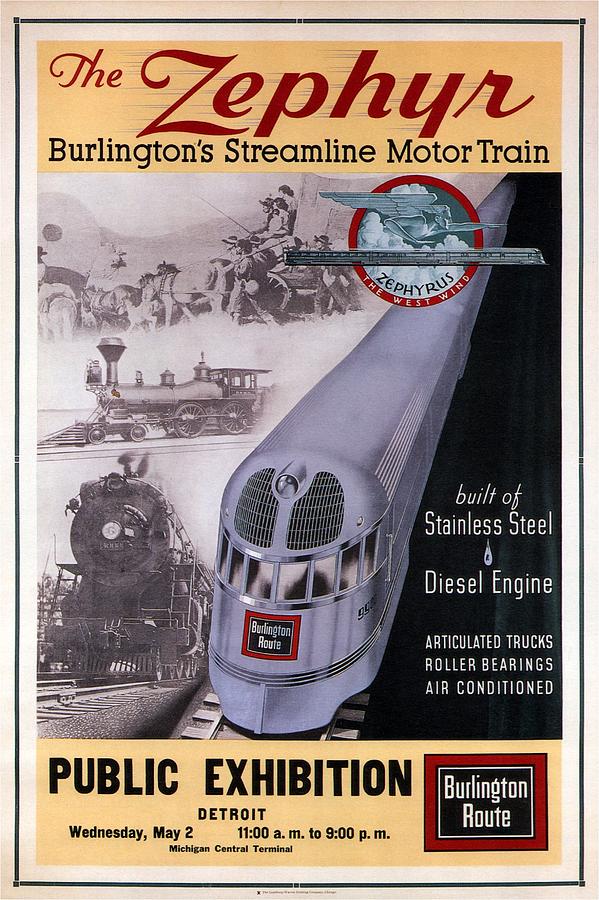This vintage poster, printed on beige paper with a thin black outline, prominently features "The Zephyr, Burlington's Streamline Motor Train" in a yellow horizontal strip at the top. Below this headline, in the center, there is a grey illustration of the modern silver train, viewed from a top-down perspective, with the Burlington Route logo at the front. To the left of the train illustration, there is a series of black-and-white photographs: the top photo shows people riding bullock carts, the middle photo features an older steam engine train, and the bottom photo displays a more modern early 1900s train, all capturing the evolution of transportation. On the right side of the train illustration, text in a black area lists the train's features: "Built of stainless steel, diesel engine, articulated trucks, roller bearings, air-conditioned." Another yellow horizontal strip at the bottom of the poster announces a "Public Exhibition, Detroit, Wednesday, May 2, 11:00 am to 9:00 pm, Michigan Central Terminal, Burlington Route."